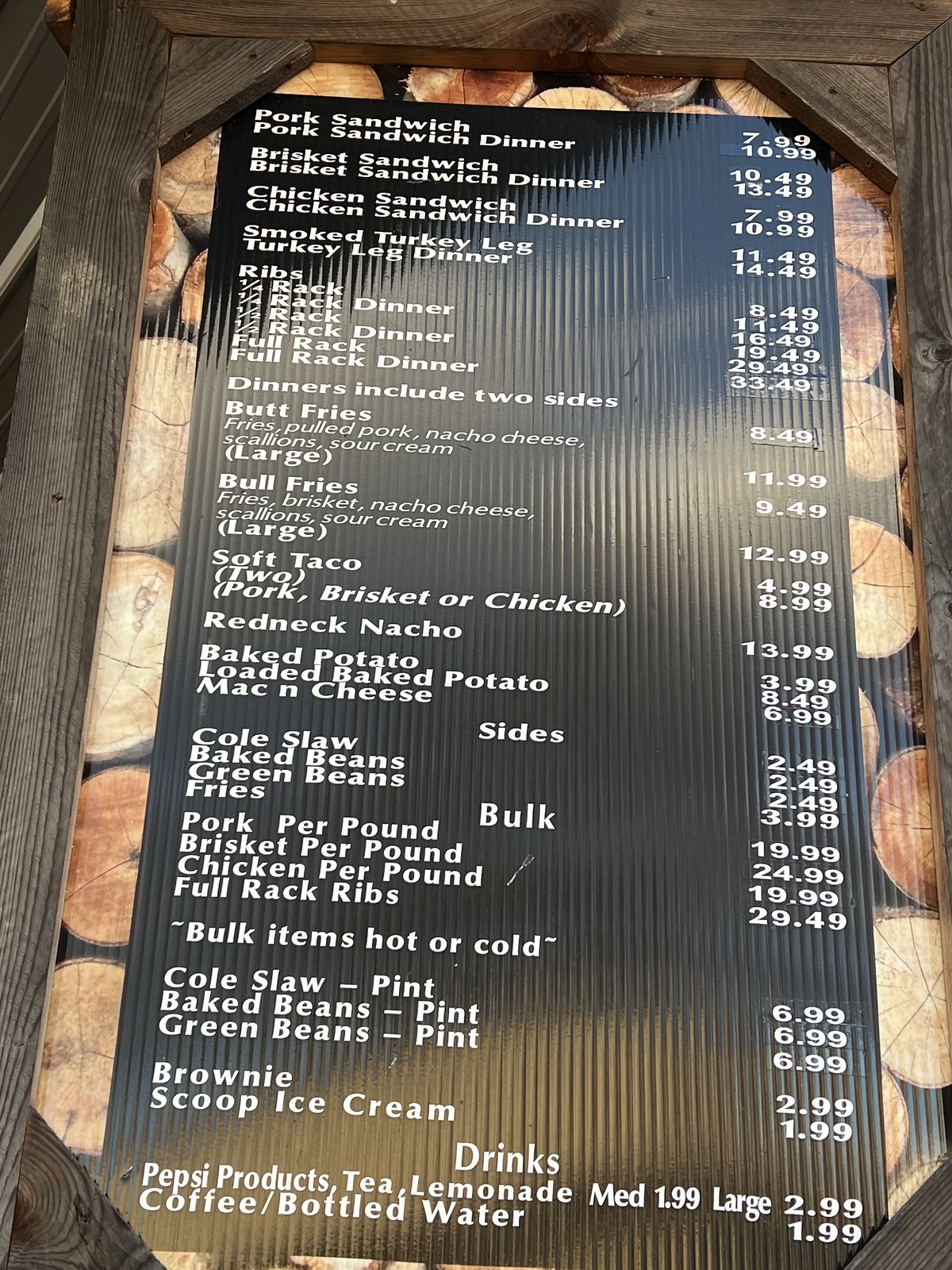This vertical image captures a detailed menu elegantly framed in weathered barnwood, showcasing a rustic aesthetic. The menu, black with crisp white lettering, stands prominently against a backdrop of round, coin-like images decorated with small black segments and golden-brown hues. These coin-like elements, likely several inches in diameter, blanket the entire frame's interior, adding a unique texture and visual interest.

The menu meticulously lists a variety of offerings, starting with sandwiches. At the top, you find pork sandwiches for $7.99, available as a dinner with sides for $10.99. Following are brisket sandwiches priced at $10.49, with a dinner option for $13.49. Chicken sandwiches are listed at $7.99, with the dinner version for $10.99. Additionally, smoked turkey legs are available for $11.49 or as a dinner for $14.49. 

The menu also features various sizes of ribs. Dinners include two sides, with options such as butt fries, bull fries, soft tacos, redneck nachos, baked potatoes, and coleslaw. Meat is available in bulk: pork per pound at $19.99, brisket per pound at $24.99, and chicken per pound at $19.99. A full rack of ribs costs $29.49. Bulk items can be served hot or cold, with sides like coleslaw, baked beans, and green beans priced at $6.99 per pint.

For dessert, a brownie is available for $2.99, with an option to add a scoop of ice cream for an additional $1.99. The menu concludes with a selection of drinks including Pepsi products, tea, and lemonade, with mediums priced at $1.99 and larges at $2.99. Coffee and bottled water are each $1.99.